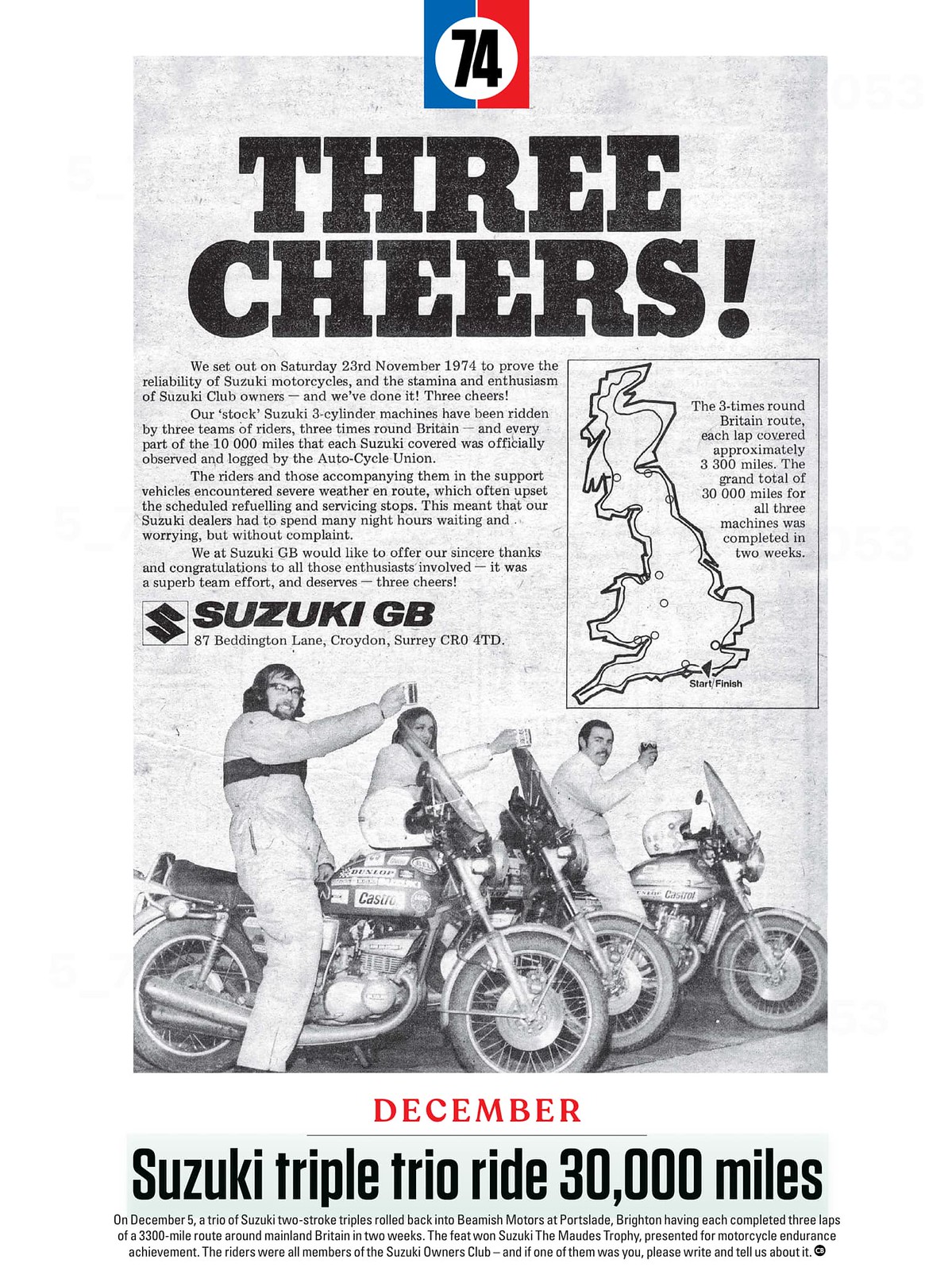The image depicts a vintage black-and-white advertisement for Suzuki, prominently displaying a logo at the top center, featuring a divided square with blue on the left and red on the right, and a white circle containing a black "74". Below the logo, in large, bold black font, is the headline "Three Cheers!" The ad celebrates a significant achievement dated Saturday, November 23, 1974, where Suzuki set out to demonstrate the reliability of their motorcycles and the endurance of their club members. 

Three teams of riders, each on a stock Suzuki three-cylinder machine, successfully completed a grueling 10,000-mile journey around Britain, officially monitored and logged by the Auto Cycle Union. Despite facing severe weather that disrupted planned refueling and maintenance stops, the Suzuki dealers provided unwavering support.

On the left, the ad features detailed text recounting the journey and expressing Suzuki GB's gratitude to all participants. On the right, there is a vertical rectangular box with a map of Great Britain showing the 3,300-mile route completed three times for a total of 30,000 miles in two weeks. 

At the bottom, an image showcases three motorcyclists – two men and one woman – each on a Suzuki bike adorned with Castrol, Dunlop, and other sponsorship logos. They are raising mugs in celebration, with the central rider being a woman. Below this image, the text "Suzuki Triple Trio Ride 30,000 miles" is prominently displayed, highlighting the event's completion on December 5th and the subsequent awarding of the MOTS trophy for motorcycle endurance. The ad concludes with an invitation for former participants to share their experiences.

In summary, this nostalgic advertisement glorifies a remarkable endurance feat, demonstrating the exceptional performance of Suzuki motorcycles and the dedication of their riders.